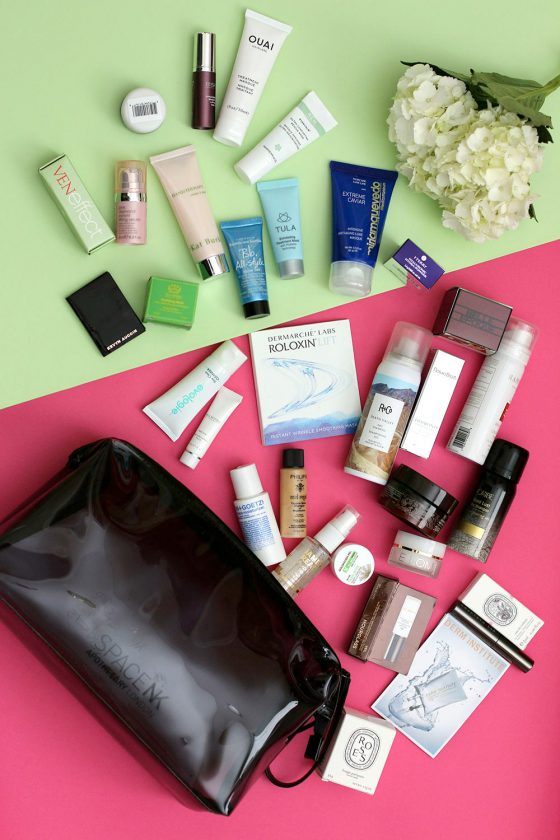In the image, a pink and green table serves as the backdrop for a meticulously organized display of beauty products. Dominating the table is a black makeup bag, identified by its label, Space NK. Surrounding the bag are its neatly arranged contents, which include various lotions, sprays, and cosmetics. Notable brands featured among the 12 to 15 items include a square container labeled Riloxin, a small white lotion container from OUAI, and a petite green box from Venn. In the top right corner of the picture, a delicate white flower adds an elegant touch to the composition.